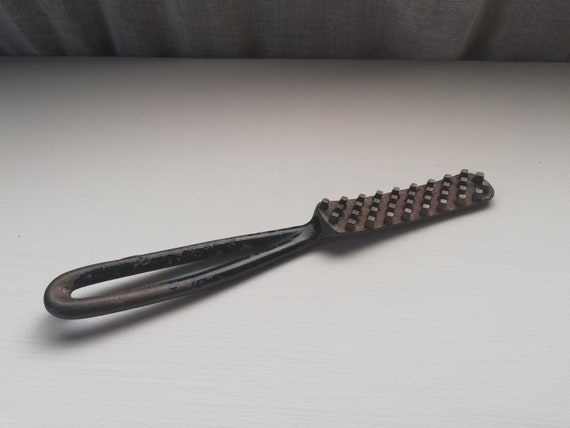In the image, a dark gray, possibly cast iron, tool is placed on a plain white counter against a tin wall with grooves. The tool has a long, longitudinal handle that forms a loop at one end, resembling the eye of a needle, and extends into an open rectangular structure at the other end. This rectangular tip is characterized by a series of small, square, metal prongs or tines that are thicker than those typically found on a brush. The tool exhibits signs of an old black powder coat finish that has rubbed off in many places, revealing an underlying reddish-brown hue indicative of rust. The metal appears worn and aged, suggesting it might be used for creating indentations or marks, though its exact purpose remains unclear.